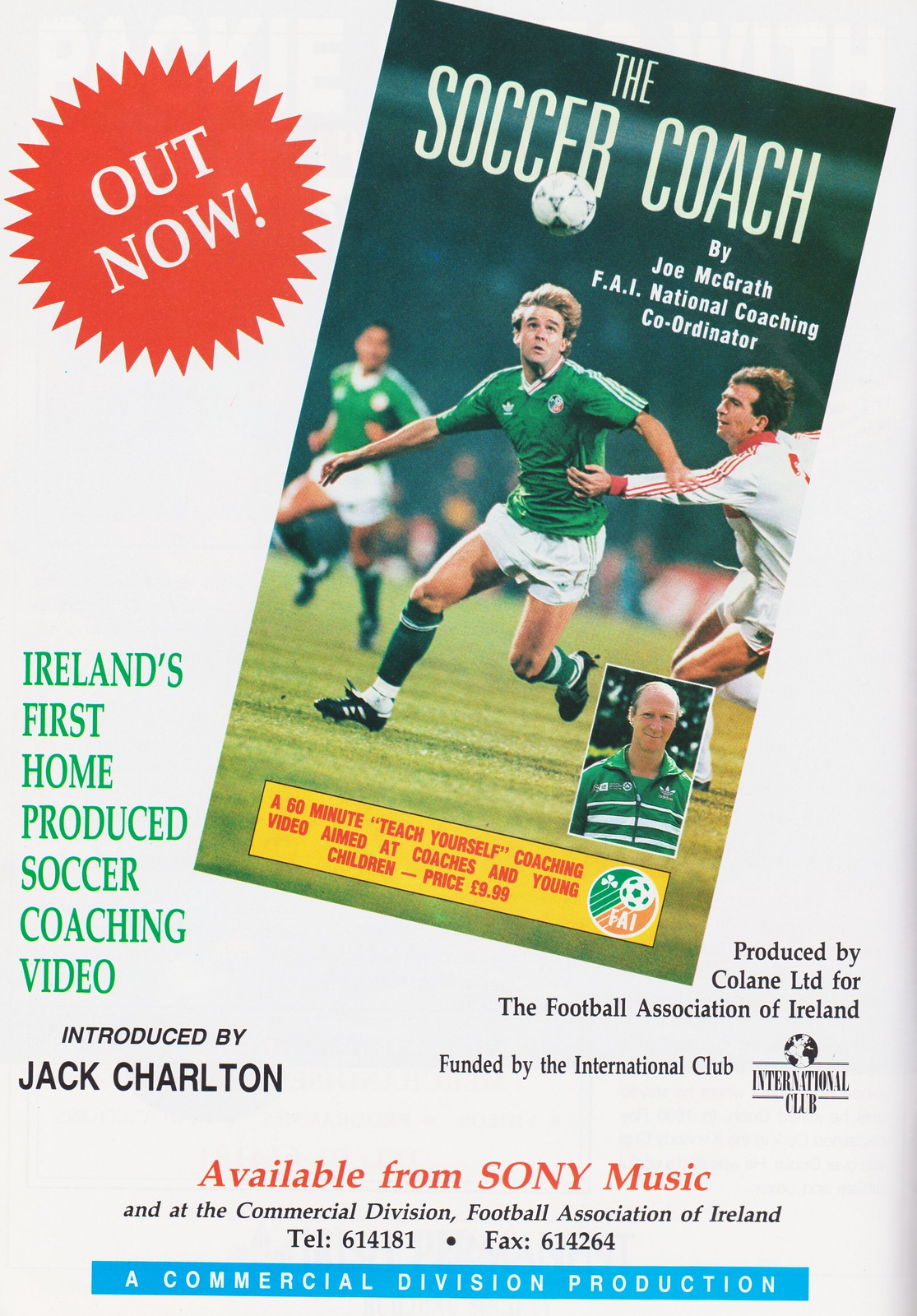This detailed advertisement image is for a coaching video titled "The Soccer Coach" by Joe McGrath, the FAI National Coaching Coordinator. The central photo captures the intensity of a soccer match featuring three players: two in green jerseys and white shorts, and one in a white jersey with red stripes. The player in the middle, donning the green jersey and black shoes, is being pursued by the opposing player in white, who has his hand on the green player's body. A soccer ball is suspended in mid-air above them, adding to the action.

Text elements on the advertisement highlight the video's details. A yellow box prominently states: "A 60-minute teach-yourself coaching video aimed at coaches and young children priced at £9.99." Above this box, a round graphic with the letters FAI, a three-leaf clover, and a soccer ball signifies the Football Association of Ireland's endorsement.

On the left, an orange and green sticker reads "Out Now" and "Ireland's first home-produced soccer coaching video" in black text. It mentions the video's introduction by Jack Charlton and notes its production by Colang Limited for the Football Association of Ireland, funded by the International Club. There's a logo for the International Club, featuring gold and red colors.

The bottom right corner of the image has an insert of Joe McGrath's photo. He is a balding white man wearing a gray, white, and green zip-up jacket with white stripes.

Additional information in smaller text details availability from Sony Music and the Commercial Division of the Football Association of Ireland, with contact details provided. The ad copy states: "Available from Sony Music and at the Commercial Division Football Association of Ireland, tel. 614-181, fax 614-264."

This colorful and comprehensive advertisement appears to be the back cover of a sports program booklet, effectively promoting a valuable resource for soccer coaches and young players alike.